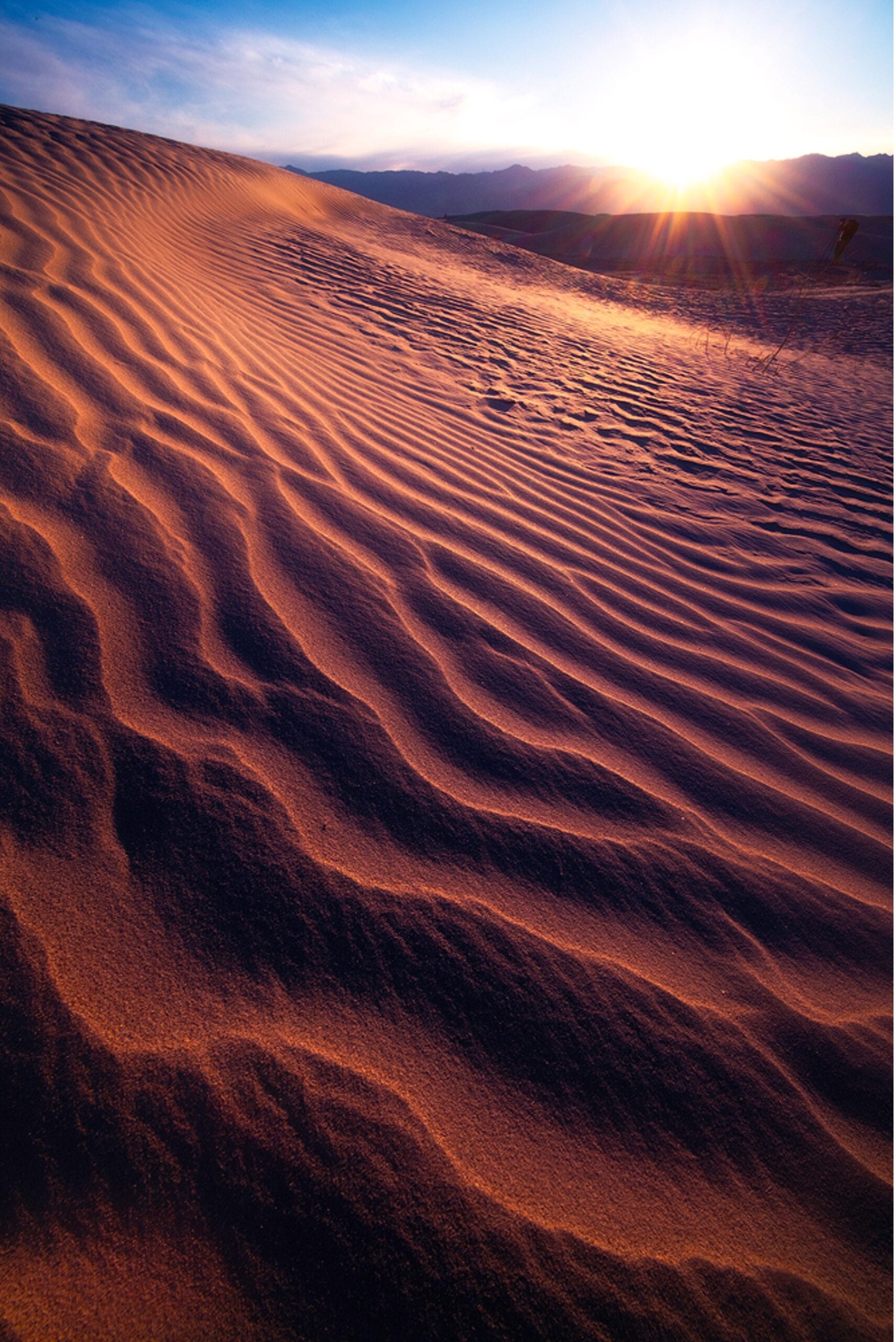A detailed photograph captures a captivating desert landscape during sunset. The foreground is dominated by a large sand dune that starts from the bottom of the image and rises toward the upper left corner, creating an elegant arch before sloping down towards the middle right. The dune's surface is intricately rippled, resembling waves caused by the wind, and the sand color ranges from orange to brown. Notable waves or ridges of sand stretch horizontally from the upper left to the middle right, creating a dynamic and textured pattern across the lower half of the image.

In the distance, at the upper right, several mountain peaks or possibly more sand dunes can be seen. Behind these peaks, darker silhouettes of additional mountains appear faintly against the horizon. Above them stretches a line of dark gray clouds, adding depth to the scene. The upper part of the image transitions from a white to blue gradient sky, dotted with light, wispy clouds.

The sun is positioned just above the horizon on the right side of the image, casting a bright, almost blinding light that creates a warm, yellow glow over the distant landscape. The sun's rays illuminate the dune, enhancing the orange hue and highlighting its textured surface. The overall composition captures the serene yet majestic beauty of the desert at sunset.